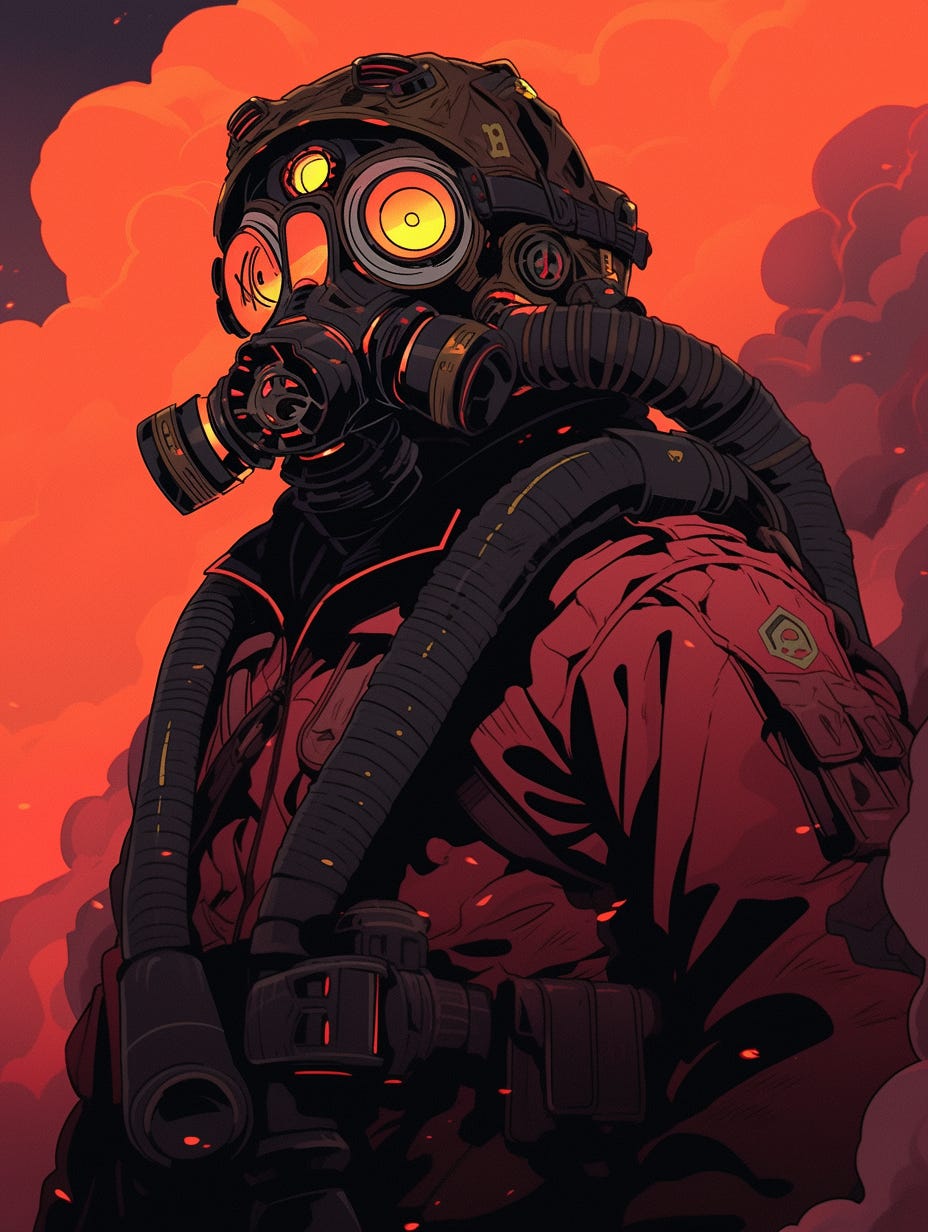This is a highly detailed, ominous drawing of a soldier, possibly taken from a comic book or video game. The image is dominated by dark browns, oranges, and reddish-purple tones, creating a foreboding atmosphere. The soldier is depicted in a three-quarter view, facing left, with only the upper torso visible. 

He is wearing an elaborate gas mask helmet that completely obscures his face. The mask is black with orange and yellow round goggles and an orange dot in the center of the forehead. Tubes emerge from the sides of the mask, wrapping around his shoulders and chest, extending towards his back. His attire is a maroon or burgundy uniform, accented by black straps, an equipment belt, and a green patch on one shoulder.

The background features orange and slightly purplish clouds of smoke, enhancing the dramatic effect of the scene. The overall dark foreground and vivid background colors further emphasize the soldier's menacing presence. The letter "B" can be seen on the side of his helmet, adding a touch of mystery to his identity.